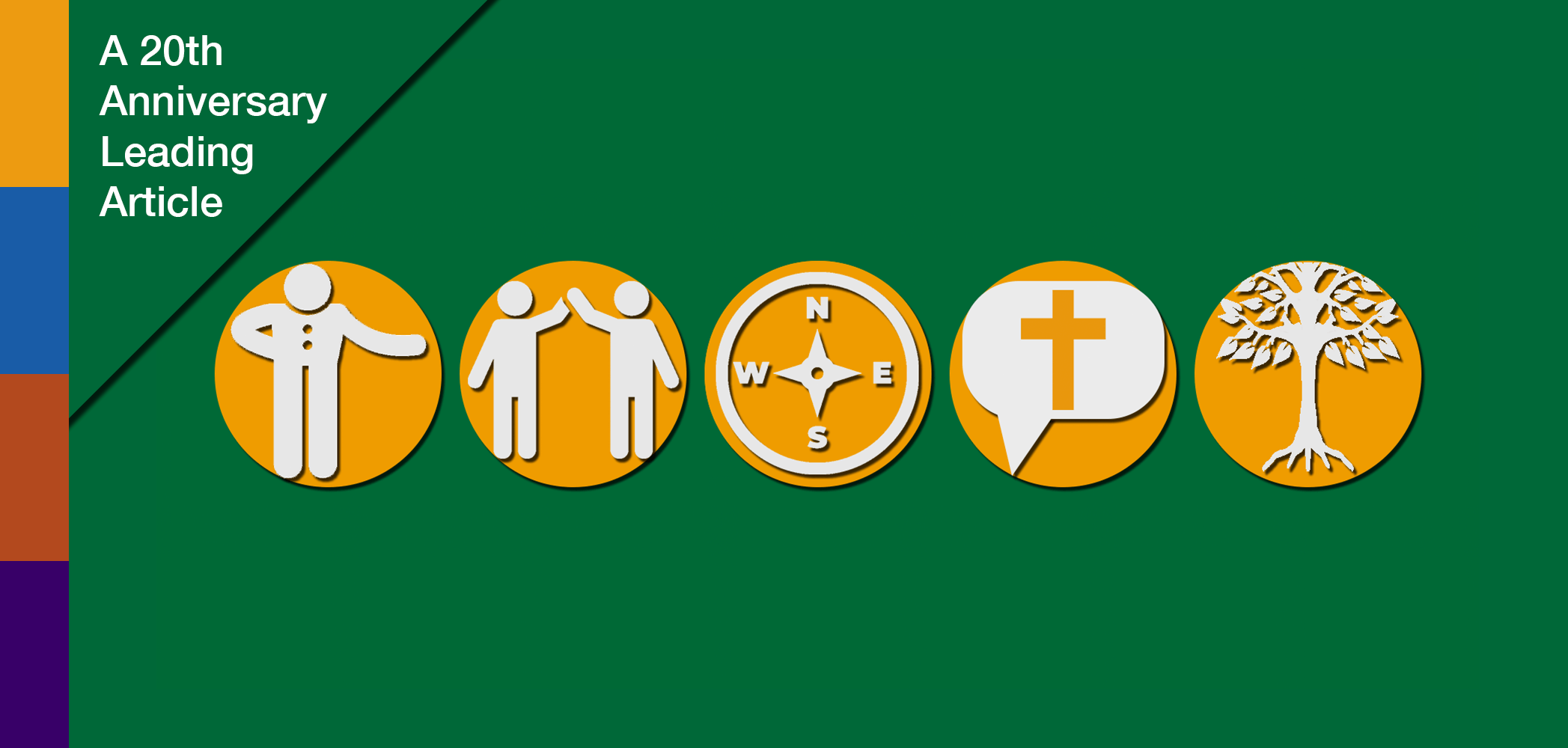The image presented is an illustrative advertisement with a distinctly green background. Dominating the left edge, there is a vertical stripe composed of four stacked, thin rectangles in the colors yellow, blue, red, and purple from top to bottom. Adjacent to this colorful stripe, in the top left corner, white text reads "20th Anniversary Leading Article." In the center of the image, five golden-yellow circles are aligned horizontally, each featuring a distinct white silhouette symbol. From left to right, these symbols depict: a man leaning forward with his arms positioned distinctively, two people high-fiving, a compass marked with directions, a speech bubble with an 'X' inside, and a tree in full bloom. Each of these symbols is finely outlined in black to enhance their visibility against the golden circles. Overall, the poster effectively uses a combination of green and golden tones with contrasting white symbols and text to create a visually engaging advertisement celebrating a significant milestone.